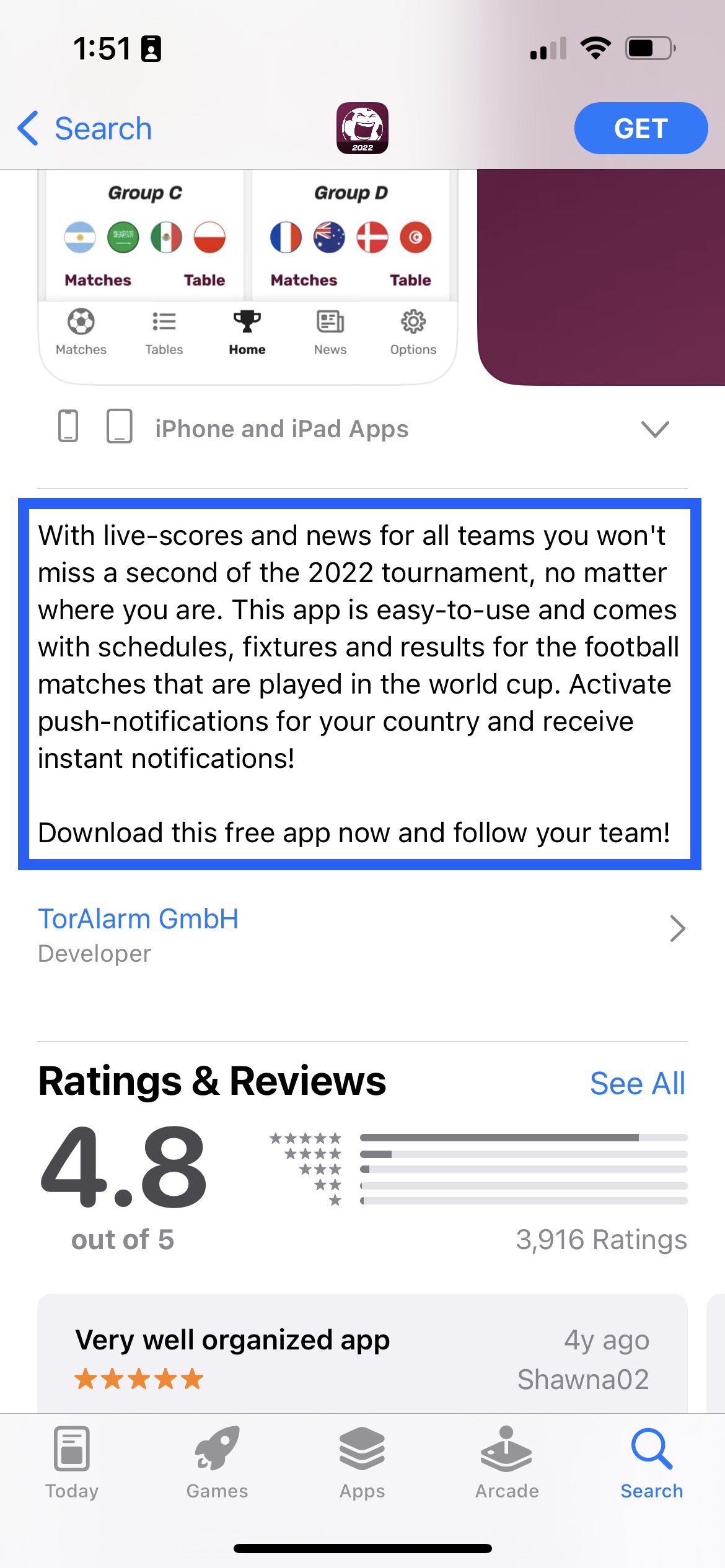A smartphone screen displays an app related to a soccer tournament. In the top left corner, the screen shows the time "1:51" and a battery icon indicating it is about half full alongside a two-bar signal strength indicator. Below this is a clickable blue word indicating "search" and an option to "go back." 

At the center of the screen, there's a logo resembling a soccer ball with a face on it, though the text is not entirely clear. To the right of the logo, there's a blue button labeled "Get." 

The main section of the screen features headings for Group C and Group D, likely representing groups from the tournament. Each group includes clickable options for "matches" and "tables." The groups appear to include countries, presumably one group from South America and one from Europe. 

Further down, additional buttons are labeled "matches" (accompanied by a soccer ball icon), "tables" (with line icons), "home," and several other options. Dominating the middle section is a large blue box with promotional text: "With live scores and news for all teams, you won’t want to miss a second of the 2022 tournament, no matter where you are."

Below this promotion, the app's ratings and reviews mention a high user rating of 4.8 out of 5, based on nearly 4,000 reviews, indicating it is well-regarded. The first review visible praises the app's organization, making it clear that this app is a useful tool for soccer enthusiasts.